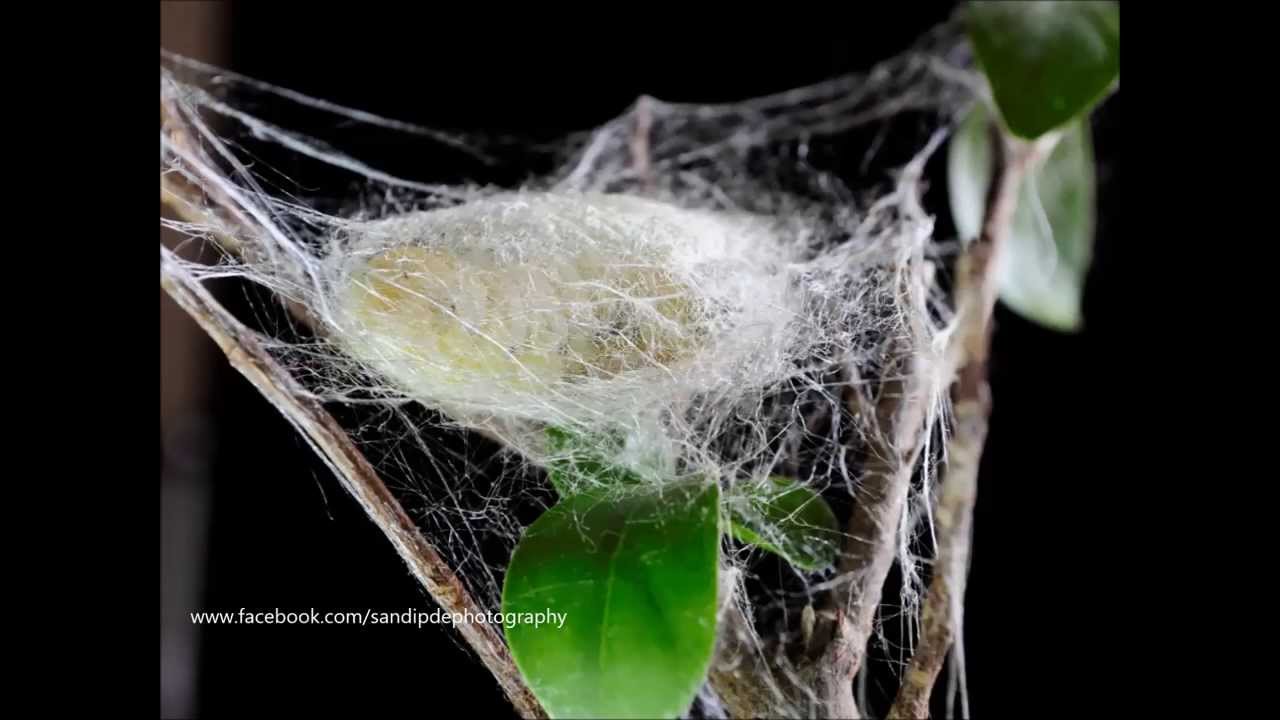The image, credited to the artist via the watermark www.facebook.com/sandipdephotography, is a highly detailed macro photograph featuring a meticulously crafted spider web nestled among twigs or stems of a plant. The web radiates from a central light yellow cocoon, extending intricately towards the twig edges. The web formation is conical, tapering into a tight, round nest-like structure that integrates seamlessly with the surrounding branches. A bright green leaf is prominently displayed front and center, appearing to support the weight of the web. Set against a dark black background, the bright colors of the cocoon, web, and foliage stand out vividly. Every detail, from the web’s delicate threads to the plant’s vibrant elements, is captured with striking clarity, showcasing the spider's intricate craftsmanship and the beauty of this natural phenomenon.